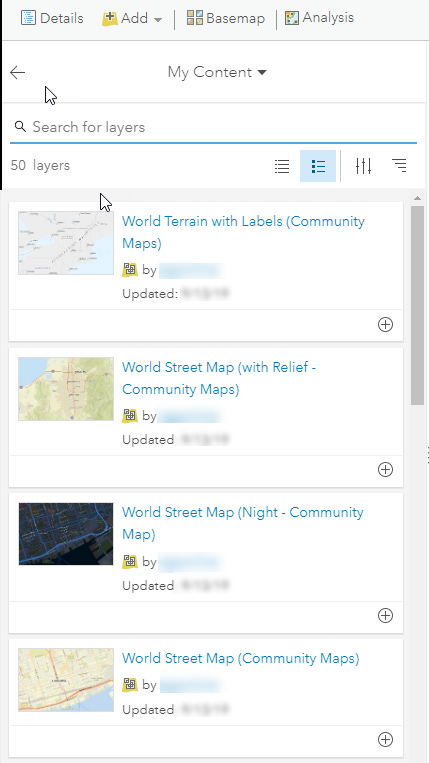A screenshot taken from a cell phone displays a detailed view of an app interface. At the top of the screen, there are tabs labeled "Details," "Add," "Base Map," and "Analysis." Below this, a horizontal section features a left-pointing arrow and a labeled strip reading "My Content" with an arrow pointing downwards. The section beneath it shows a search bar labeled "Search for layers" with a note indicating "50 layers." Four icons are present, with the second one from the left being selected.

Further down, a list of map layers is visible. First on the list is "World Terrain with Labels, Community Maps," followed by a blurred author and update information, ensuring privacy. The subsequent layers include: "World Street Map with Relief, Community Map," "World Street Map Night, Community Map," and at the bottom, "World Street Map (Community Maps)." Each of these map layers is accompanied by a plus sign located in the lower right corner of their respective sections.